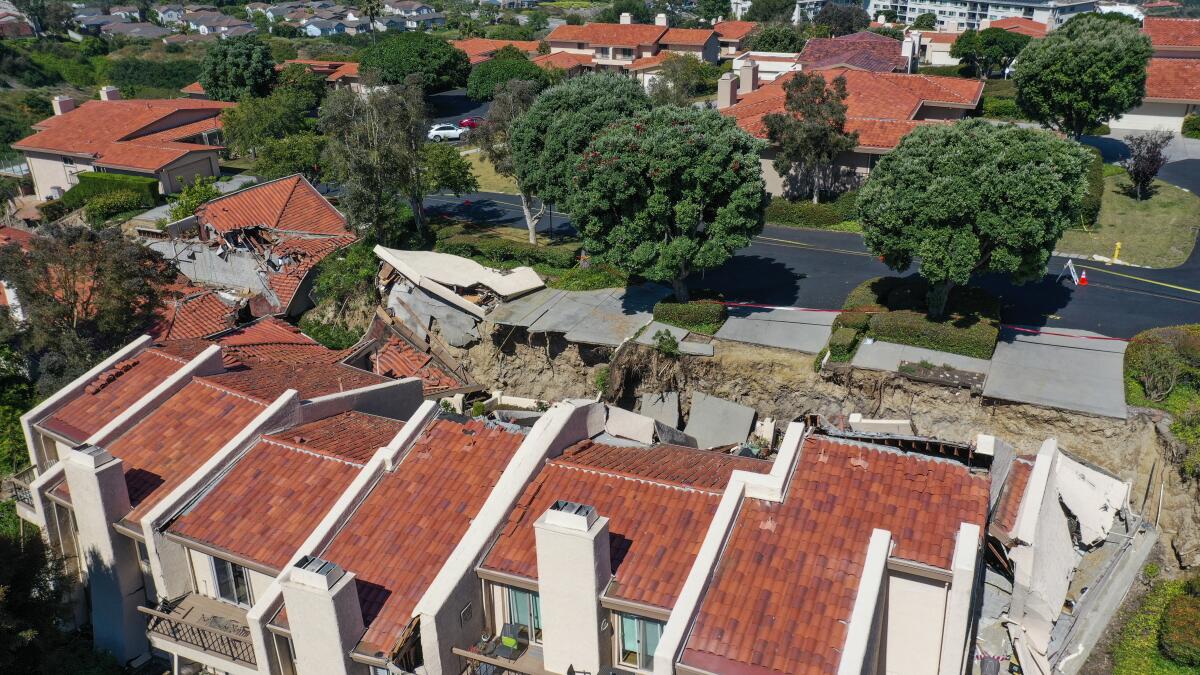This color aerial photograph, likely taken by a drone, vividly captures the aftermath of a devastating sinkhole that has engulfed multiple homes in a residential area. The image reveals a striking contrast between the destroyed and intact structures. In the center of the frame, a massive sinkhole runs diagonally from left to right, causing several duplexes and terraced homes with white stucco walls and red tile roofs to collapse into a huge chasm lined with broken concrete and debris.

The destruction is evident: roofs are shattered, and buildings crumbled, leaving a strip of devastation amidst an otherwise orderly neighborhood. While some multi-story homes remain intact, the ones directly affected by the sinkhole have been almost entirely obliterated.

A well-paved road, marked with traffic cones and red tape, bisects the scene and highlights the damaged area, emphasizing the urgent need for repair. Green, bushy trees topped with leaves stand in stark contrast to the disaster, lining the road and dotting the landscape. In the background, larger apartment buildings and clusters of grey-roofed houses appear undisturbed, framing the calamity with a sense of normalcy.

Details abound: chimneys and balconies adorn the partially visible homes clipped by the frame, a solitary white car is parked in the distance, and red markings are noticeable on some trees. The bright daylight casts an unforgiving light on the scene, demarcating the area of ruin from the untouched sections of the neighborhood, and painting a vivid tableau of nature's unexpected fury.